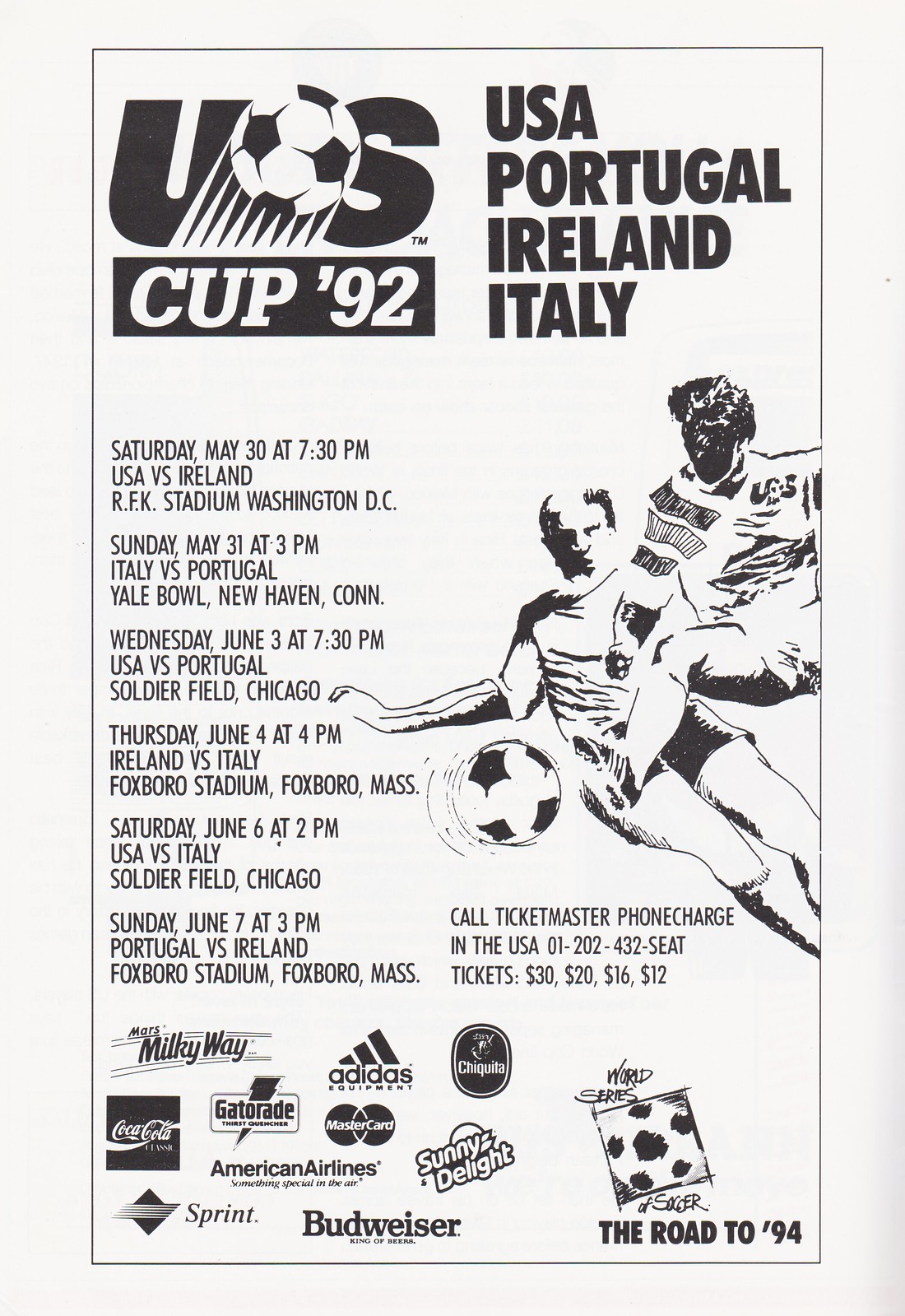The black-and-white image, styled like a vintage print publication, is an informative flyer for the U.S. Cup 92, featuring the national teams of the USA, Portugal, Ireland, and Italy. The top section prominently displays "USA, Portugal, Ireland, Italy" in bold, stacked lines, with the event title "U.S. Cup 92" on the left, incorporating a logo depicting a soccer ball. The flyer lists all match details vertically, with specifics on dates, times, and venues: USA vs. Ireland on Saturday, May 30th at 7:30 p.m. at RFK Stadium in Washington, D.C.; Italy vs. Portugal on Sunday, May 31st at 3 p.m. at Yale Bowl in New Haven, Connecticut; USA vs. Portugal on Wednesday, June 3rd at 7:30 p.m. at Soldier Field in Chicago; Ireland vs. Italy on Thursday, June 4th at 4 p.m. at Foxborough Stadium in Foxborough, Massachusetts; USA vs. Italy on Saturday, June 6th at 2 p.m. at Soldier Field in Chicago; and Portugal vs. Ireland on Sunday, June 7th at 3 p.m. at Foxborough Stadium in Foxborough, Massachusetts. The flyer further provides details for ticket purchases, directing to Ticketmaster with pricing options of $30, $20, $16, and $12, alongside a contact phone number, 01-202-432-SEAT. The bottom of the flyer showcases logos of numerous sponsors including Milky Way, Coca-Cola, Gatorade, Adidas, MasterCard, American Airlines, Sprint, Budweiser, Sunny Delight, and Chiquita. The right side of the flyer features outlined illustrations of two soccer players in action. The overall design is framed by a black border, giving it a striking and organized appearance.